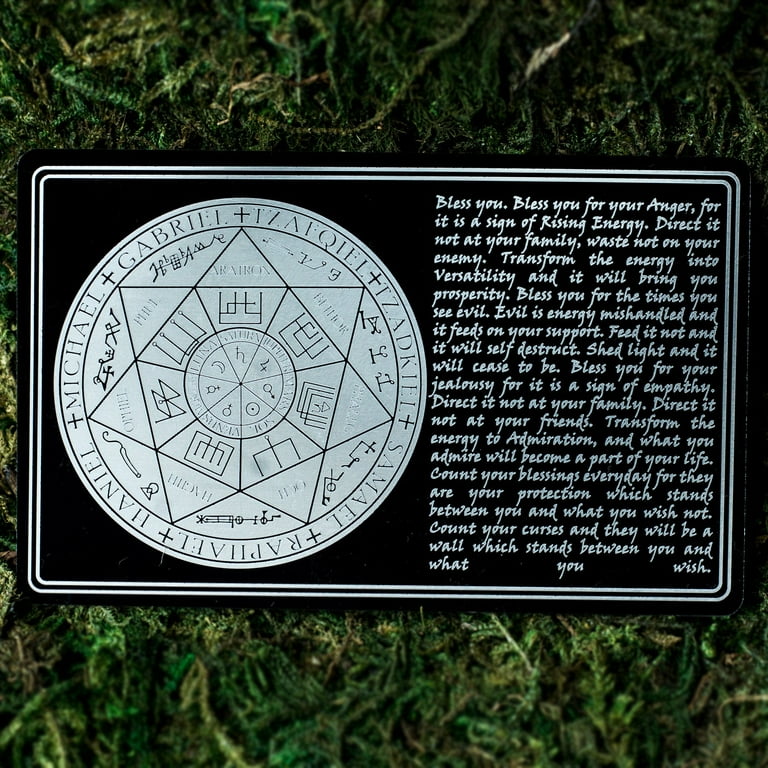The photograph features a square image, approximately six inches by six inches, depicting a black card with a silver circular emblem and text, nestled on a bed of green moss. The card, a horizontal rectangle with beveled edges, has a black background bordered by two thin silver pinstripe lines. The left side of the card showcases a prominent silver circular emblem containing geometric shapes, line drawings, and hieroglyphic-like symbols. Encircling the emblem, black text lists names separated by black crosses, including Michael, Gabriel, Tzadkiel, Samuel, Raphael, and Haniel. The right side of the card is dominated by a detailed paragraph of silver text that reads: "Bless you, bless you for your anger for it is a sign of rising energy. Direct it not at your family, waste not on your enemy. Transform the energy into versatility and it will bring you prosperity. Bless you for the times you see evil. Evil is energy mishandled and it feeds on your support. Feed it not and it will self-destruct, shed light and it will cease to be. Bless you for your jealousy for it is a sign of empathy. Direct it not at your family. Direct it not at your friends. Transform the energy into admiration and what you admire will become a part of your life. Count your blessings every day for they are your protection which stands between you and what you wish not. Count your curses and they will be a wall which stands between you and what you wish." Surrounding the card is a thin layer of green foliage, adding a natural touch to the image.